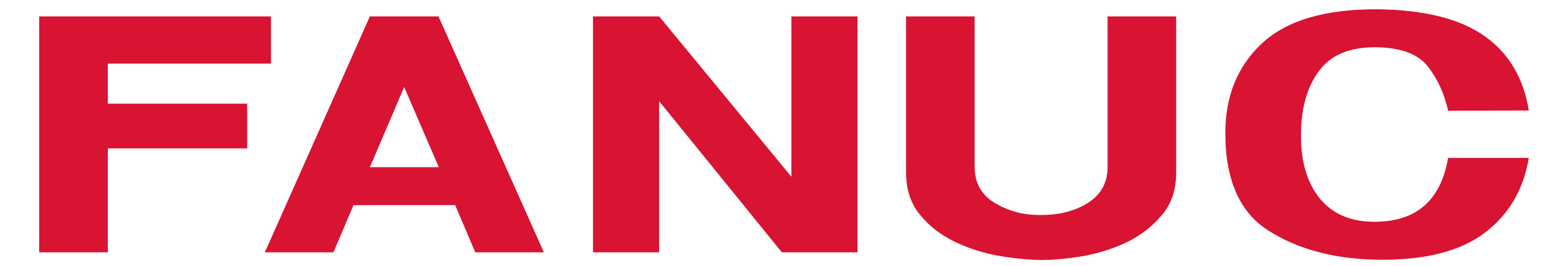This horizontal, borderless image features the bold, capital letters F-A-N-U-C, rendered in a deep red color. Set against a plain white background, the letters are large and composed of thick red lines, emphasizing their prominence. Notably, the letter 'C' stands out with its unique design: an almost closed gap creates a near-oval shape at its center, adding a touch of visual interest. The absence of any additional context or background details leaves us to surmise that FANUC is likely the name of a company.